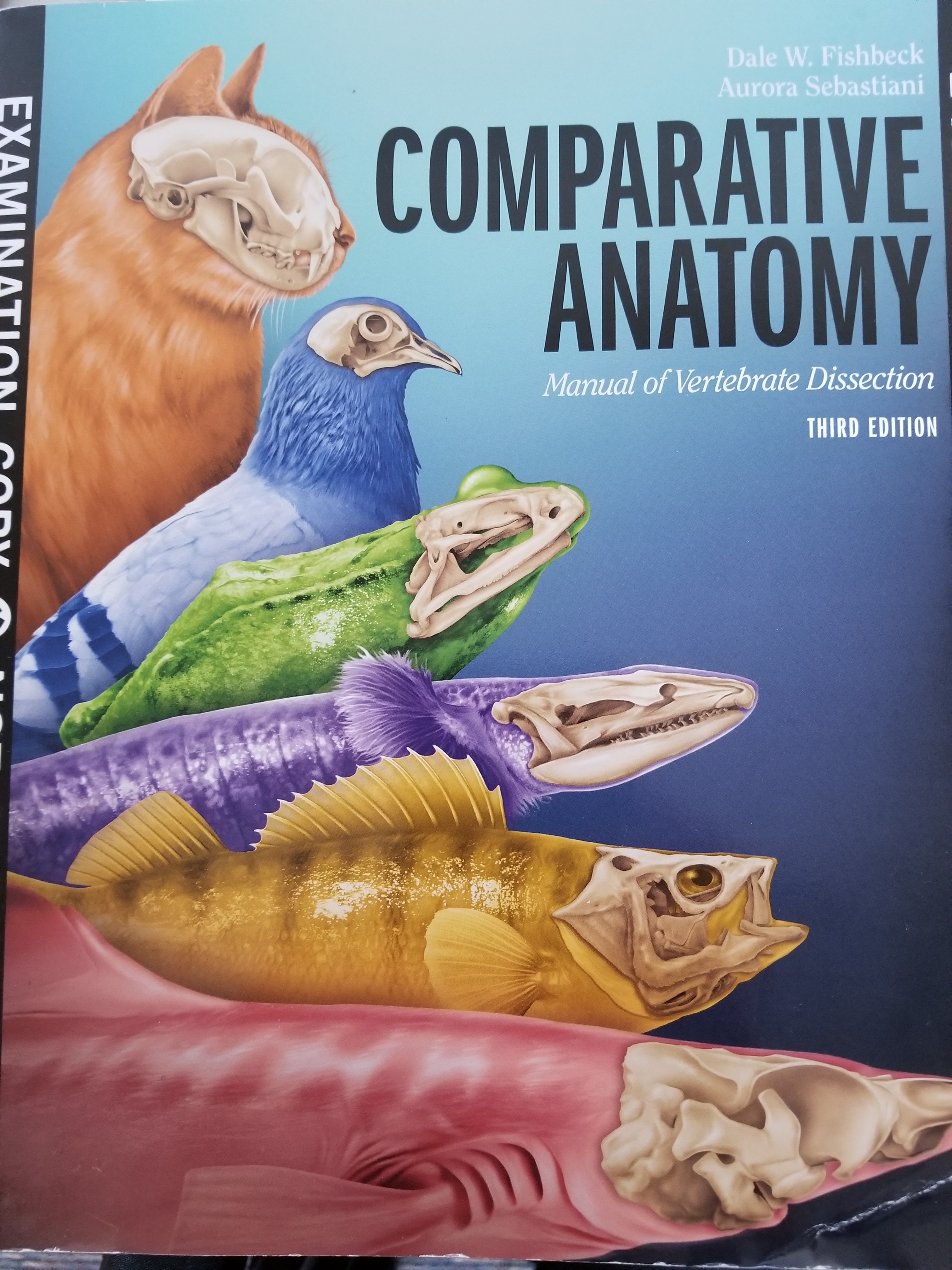The image depicts the cover of a book titled "Comparative Anatomy: Manual of Vertebrate Dissection, Third Edition," set against a blue background that transitions to a darker shade at the bottom. The authors, Dale W. Fishbeck and Aurora Sebastian E., are listed in white text at the top. The title is prominently displayed in black text to the right side of the image, with "Manual of Vertebrate Dissection" and "Third Edition" also in white text below. A black stripe in the upper left corner reads "Examination Copy" in white text. On the cover, various animals are illustrated with their skeletal structures partially exposed, including a cat at the top showing its lower body and skull, a bluebird, a frog, and three fish, each depicted with exposed skulls. The image is vertical and rectangular.